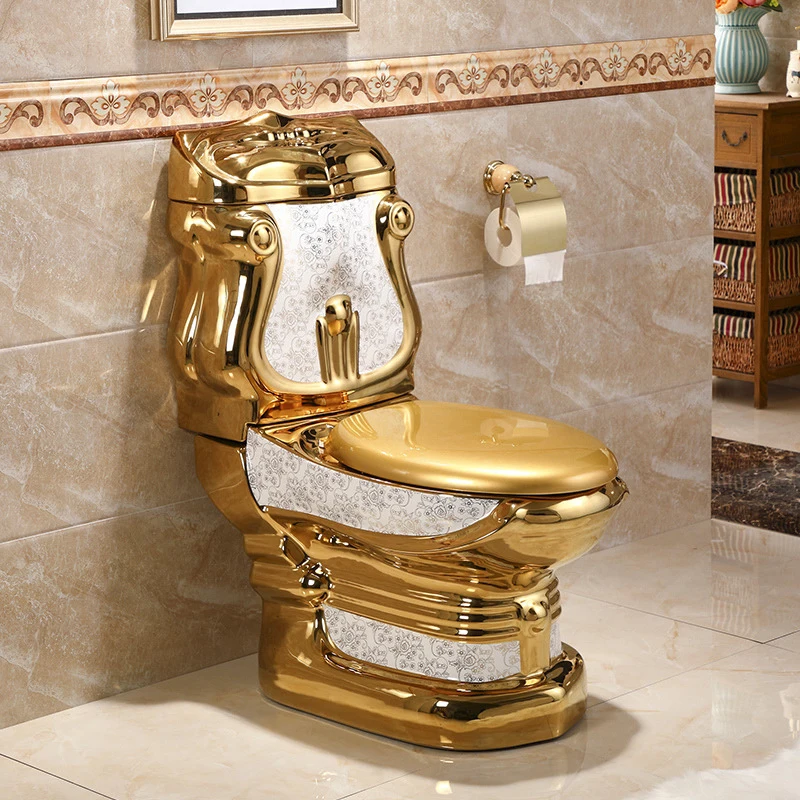The image showcases an opulent bathroom featuring a striking golden toilet that stands as the centerpiece. This lavish fixture gleams with a super shiny gold plating, covering the lid, base, and tank, which includes intricate white strip paneling adorned with black floral designs right above the base and below the seat. The front of the tank also has a white inner section with similar black floral ornaments, encircled by a gold curved inlay design. The golden toilet lid is particularly reflective, offering a mirror-like finish when down.

The bathroom itself exudes luxury, with light tan marble tiles gracing both the floor and the walls, adding to the sophisticated ambiance. The tiles are glossy and reflective, enhancing the bathroom's grandeur. Even the toilet paper holder, sitting adjacent to the toilet, is gold-plated, carrying the same extravagant theme. Above the toilet, the lower edge of a golden picture frame is visible, suggesting more opulence extends beyond the frame of the photograph. To the right, part of a wooden dresser from the adjoining room is just barely visible, hinting at the contiguous luxurious decor. This bathroom undoubtedly reflects a taste for extravagant wealth and meticulous decorative detailing.